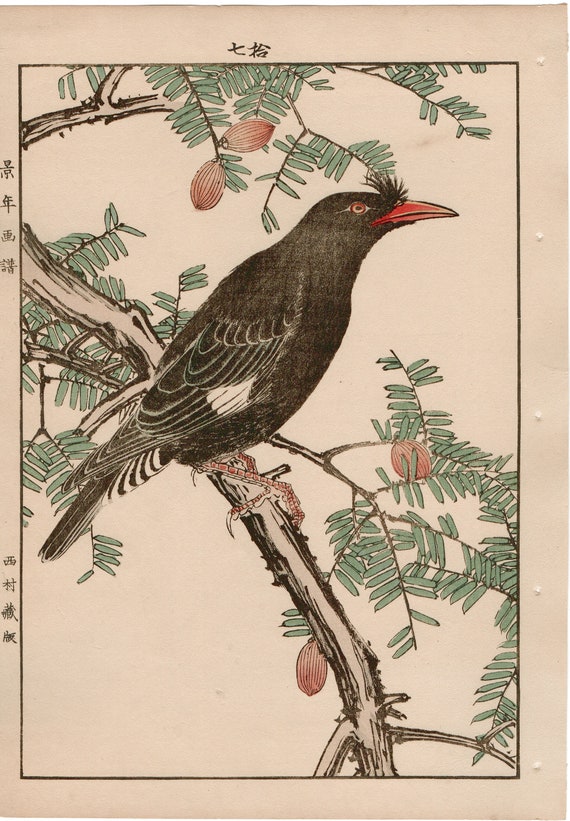The image depicts a striking black bird set against a white backdrop intricately adorned with tree branches. These branches emanate from the top center, the right, and the center left of the image, creating a natural frame around the bird. The branches are sprouting leaves reminiscent of green beans or shaved leaves and bear fruit that resemble peanuts or pecans in shape.

The bird itself is predominantly black, with a subtle touch of white on one part of its wing. Its tail features alternating bands of white and blue, or white and black plumage, adding a touch of contrast. The bird's face is accentuated by a small tuft of feathers, giving it a distinctive look. Its eye is a unique reddish-white color, while its beak stands out in red.

Adding a cultural element to the imagery, the left edge and the top of the cover display a set of Asian characters. Along the left side, there are four characters at the top and four more at the bottom. Positioned centrally at the top are two additional Asian characters, completing the visually engaging and culturally rich composition.